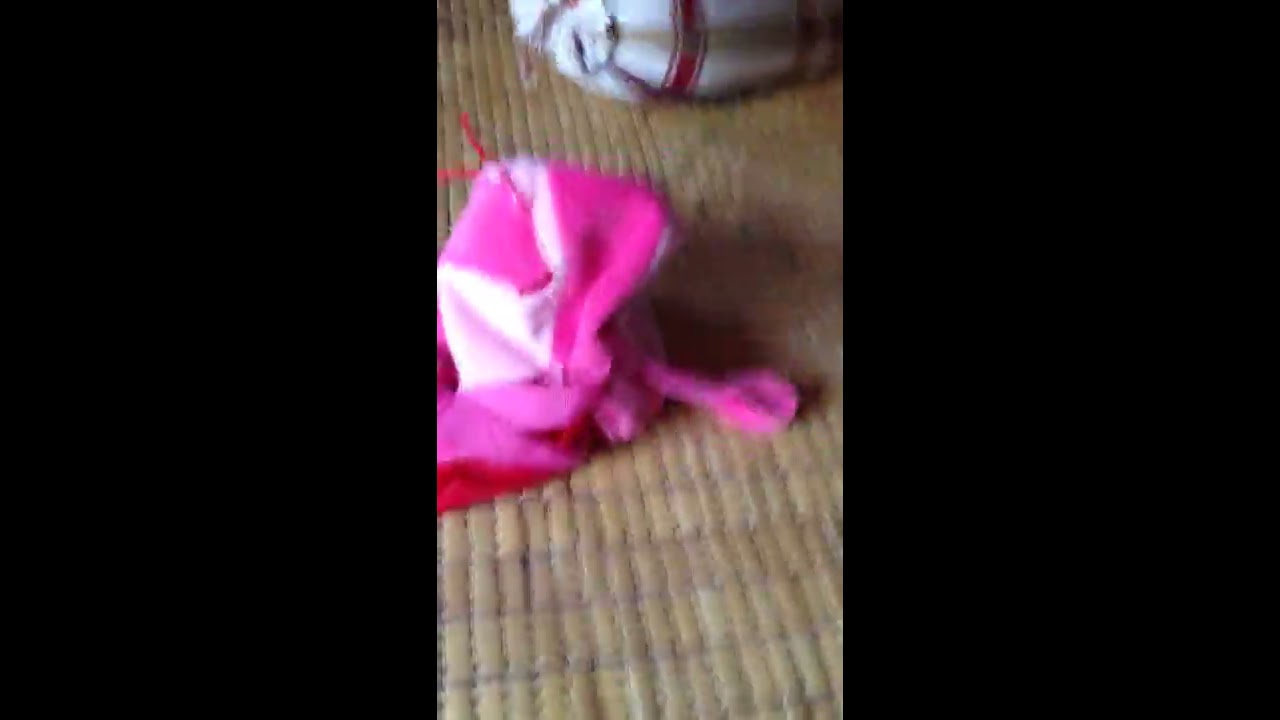This image features a blurry, difficult-to-decipher scene. The left and right thirds of the picture are completely dark, creating a stark black rectangular border. The central part of the image reveals what appears to be a woven or thatch-like flooring, brown in color and showcasing various shades. In the middle of this surface, a soft pink object lies, possibly a child's hat or a stuffed toy, exhibiting different hues of pink, light pink, and white, with two red antenna-like projections. Above this, towards the top of the image, a faint, blurry white object with red stripes is visible, potentially another piece of cloth or a hat. The objects appear strewn across the brown surface which could be flooring or a bedsheet.